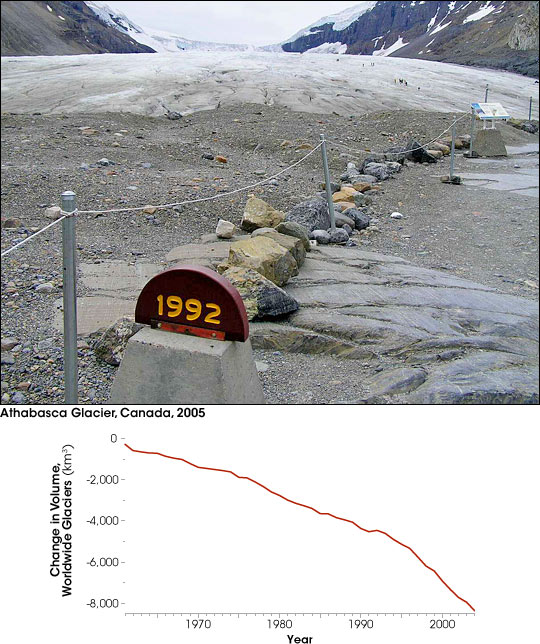This image is divided into two sections. The upper section features a photograph of the Athabasca Glacier in Canada, taken in 2005. The scene shows a desolate mountainous landscape with a row of rocks and a fenced-off area marked by silver poles connected with white rope. A small, cement pedestal prominently displays the year "1992" in red within a half-circle shape. In the background, you can see the snow-capped peaks.

The lower section of the image contains a line graph. The x-axis of the graph is labeled "Years," spanning from 1960 to 2005, while the y-axis is labeled "Change in Volume, Worldwide Glaciers (km³)," ranging from 0 to negative 8000. The red line on the graph trends sharply downwards, illustrating a significant decline in glacier volume over time. This visual representation highlights the stark effects of global warming on worldwide glaciers.